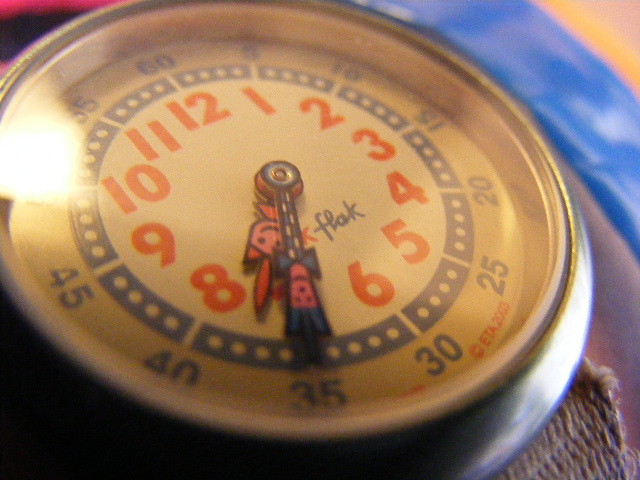This photograph features a small, vintage wristwatch with a whimsical design. The circular watch face displays numbers starting at 12 at the top, all in orange. Surrounding these numbers is a ring of blue dashes, each containing a white circle. The hour and minute hands are designed as playful cartoon characters, adding a touch of charm to the timepiece. One hand has a pink face with a smile and orange cat ears, while the other has blue hair sticking straight up and a blue bow tie. The outer perimeter of the face includes additional numbers. The image's quality suggests it was taken with an older camera, adding to the nostalgic feel of this unique, child-like wristwatch.